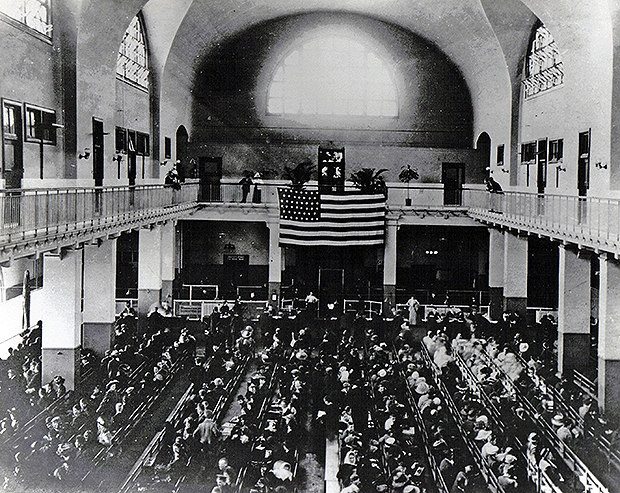This black-and-white photograph, taken many years ago, depicts a large, two-story building of indeterminate function. The image is somewhat unclear due to its age and monochrome palette, but certain details stand out. The building features an upstairs wraparound balcony with railing and a downstairs area with rows of seating, which appear to be occupied by tightly gathered people. Toward the far end of the room, one can see a series of grand columns supporting a gigantic American flag hanging between them. There are additional columns on this side of the room, enhancing the grandeur of the space. On the balcony, four individuals look downwards over the railing, observing the scene below. The overall atmosphere and architectural elements suggest that this may be a significant gathering place, possibly a church or a rotunda, fitted with pew-like seating. Other details, such as a large window providing natural light and planted trees within the establishment, add to the sense of a large, formal interior, potentially used for important communal gatherings or ceremonies.